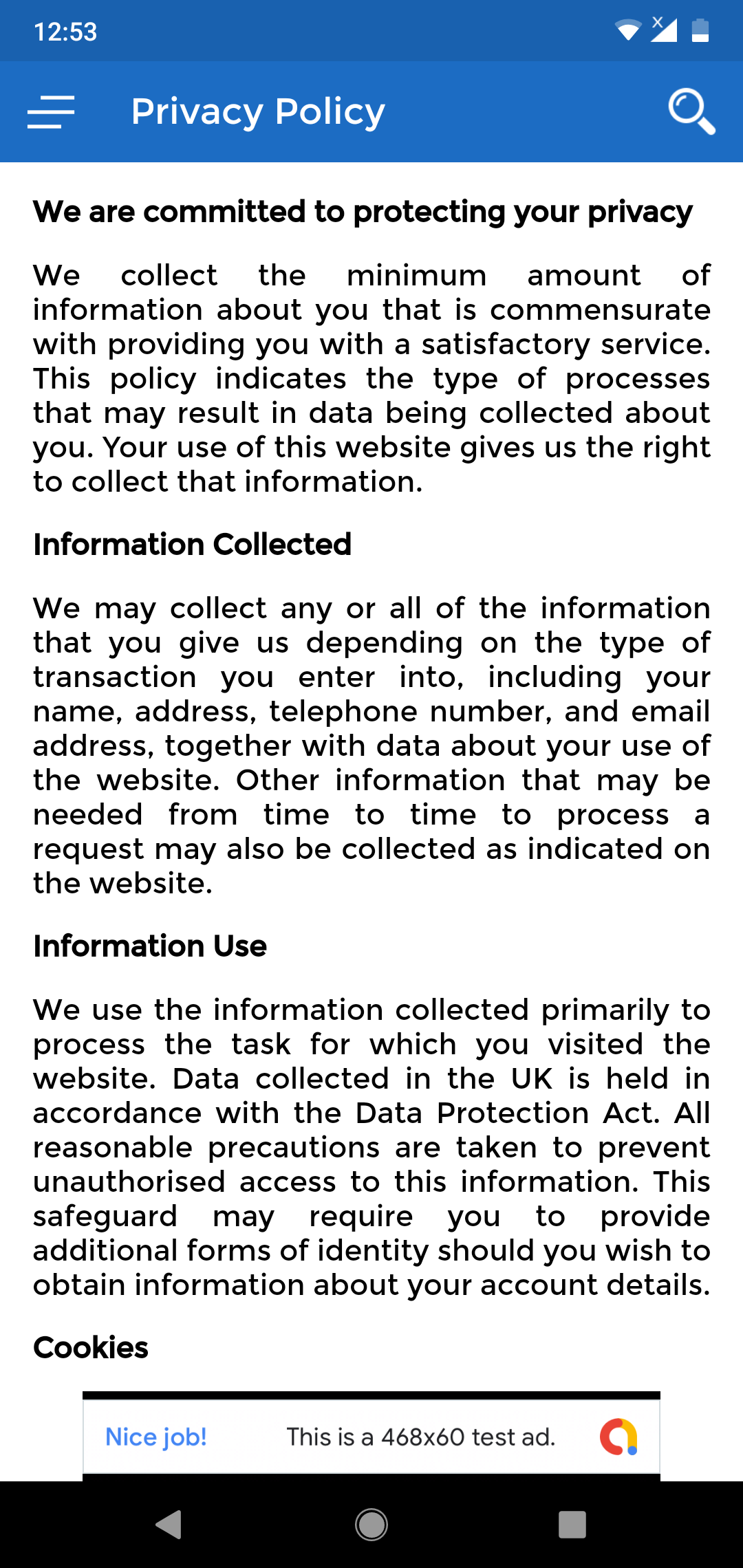The image displays a smartphone screen with several key elements. At the top left corner, the time is shown as 12:53, while the top right corner displays signal indicators for data and Wi-Fi connectivity. The cellular signal icon has an 'X' over it, indicating no service, and the battery level is quite low. Below this status bar, against a blue background, there are menu options presented as three horizontal lines stacked on top of each other on the left side, a privacy policy link in the middle, and a search icon on the right side.

Further down, on a white background, there's a detailed privacy notice. The notice emphasizes a commitment to privacy, stating, "We are committed to protecting your privacy. We collect the minimum amount of information about you that is commensurate with providing you a satisfactory service." It continues to explain the types of data collected, such as name, address, telephone number, and email address, as well as data about the user's interaction with the website. The notice assures users that collected information is used primarily to fulfill the tasks for which they visited the website, and that all data collected in the UK is handled in accordance with the Data Protection Act. Users are also informed about the precautions taken to prevent unauthorized access, including the potential requirement for additional forms of identity verification to access account details. The section concludes with a brief mention of cookies.

The lower section of the screen is marked by a black bar with unspecified text.